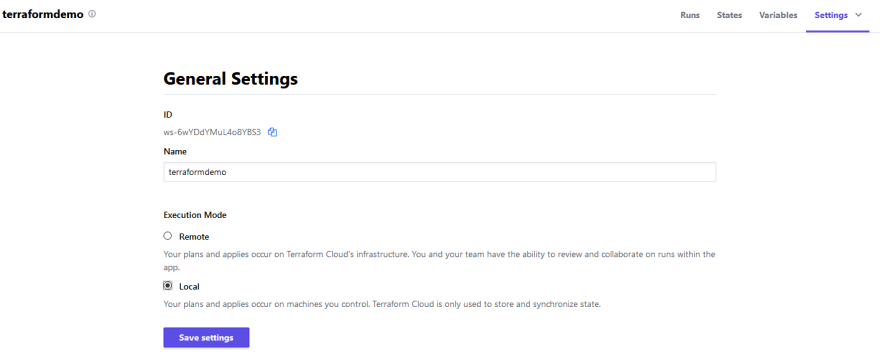The image displays a screenshot of the Terraform demo site. On the right-hand side, there are tabs labeled "Runs," "States," "Variables," and "Settings," with the "Settings" tab selected and highlighted in purple. The central part of the image shows the "General Settings" section, with "General Settings" written in bold black font, both words capitalized. Below this heading, there is a field labeled "ID" in bold black, accompanied by the ID address entered in the text box. 

Further down, there is a field for "Name" with "Terraform Demo" filled in. The "Execution Mode" section follows, providing two options: "Remote" and "Local." The description clarifies that "Remote" mode allows plans and applies to run on Terraform Cloud's infrastructure, enabling team review and collaboration on runs within the application. "Local" mode indicates that plans and applies are executed on user-controlled machines, with Terraform Cloud used solely for storing and synchronizing the state. The "Local" option is currently selected, marked by a blue outline around the selection box and dotted with black. 

At the bottom of the settings section, a sideways purple rectangle is displayed with the text "Save Settings."